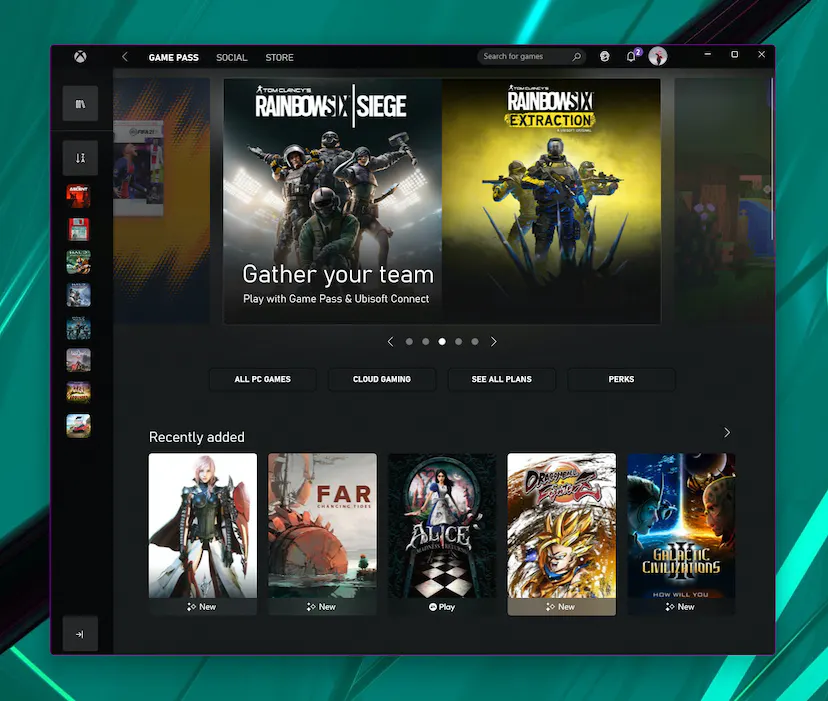A detailed view of the Xbox Game Pass app, showcasing the Game Pass tab prominently with the Xbox logo in the upper left corner. The user is logged into their Game Pass account, evident from the personalized interface. The interface displays various game titles, with "Rainbow Six Siege" prominently featured and "Rainbow Six Extraction" positioned next to it, suggesting the user has a preference for military-style, tactical team games. Other tabs available include ‘Social’ and ‘Store,’ though the focus remains on the Game Pass tab. At the bottom of the page, a 'Recently Added' section highlights the latest games available on Game Pass. Visible on the left sidebar are several previously downloaded games, indicating the user is exploring new games to download and play. The app appears to be running on a computer, though it could also be on an Xbox console.